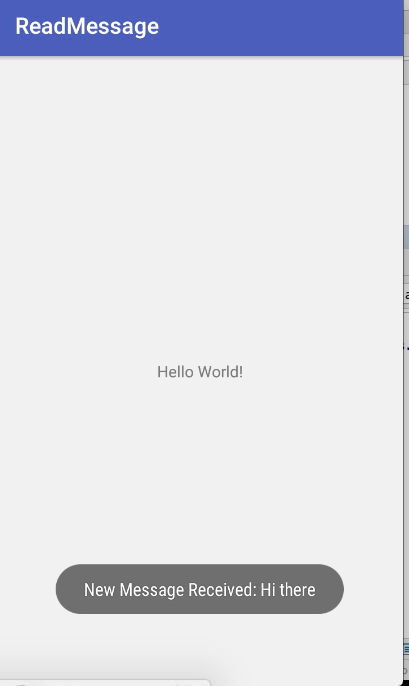The image portrays a simple, minimalistic message interface with a primarily gray background. Spanning from the upper left to the upper right corner is a prominent blue stripe featuring the text "READMESSAGE" in uppercase letters, with "READ" in bold and "MESSAGE" in regular font. The vast gray background, devoid of significant content, visually dominates the image, creating a sense of unused space.

Centrally located in small, light gray letters that blend into the background and are difficult to discern, the message "Hello world!" is displayed, which could have benefitted from a larger font size to maximize readability and space utilization. 

Towards the bottom of the image, there's a gray button with white text that reads "New Message Received" accompanied by the phrase "Hi there." This layout suggests this might be a pop-up notification or part of a larger user interface.

Additionally, from the upper right-hand side downwards, there appears to be a faint chart or patterned light gray stripes that intersect the image, possibly indicating underlying content or a background feature. This chart-like pattern is faint and barely noticeable, and it ends abruptly, giving way to a solid black section at the very bottom-right corner.

Overall, the design features a lot of empty space, with small, difficult-to-read text that detracts from its functionality and ease of use.